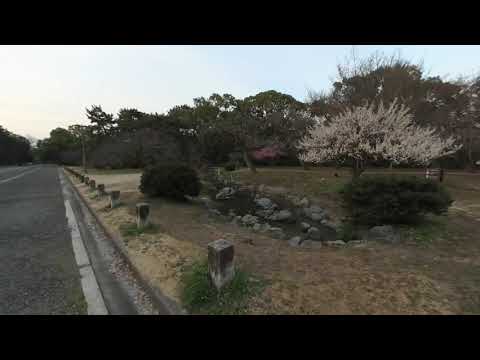This outdoor image captures a partial view of a road on the far left side with a white stripe marking its edge. Adjacent to the road are some old stone posts, hinting at where a fence might have once stood. The terrain beyond the posts features a hilly, slightly rocky area sparsely dotted with grass, shrubs, and small trees. Dominating the scene are various trees in different states: some are green, one displays vivid pink blossoms, and a prominent tree is in full white bloom. The backdrop includes a hazy sky with light blue patches and scattered clouds, implying an overcast day with limited sunshine. The absence of vehicles and illegible signage suggests a tranquil and somewhat isolated setting. This photo, characterized by its earthy tones - grays, tans, greens - and minimal contrast, appears to have been taken by someone standing by the roadside.